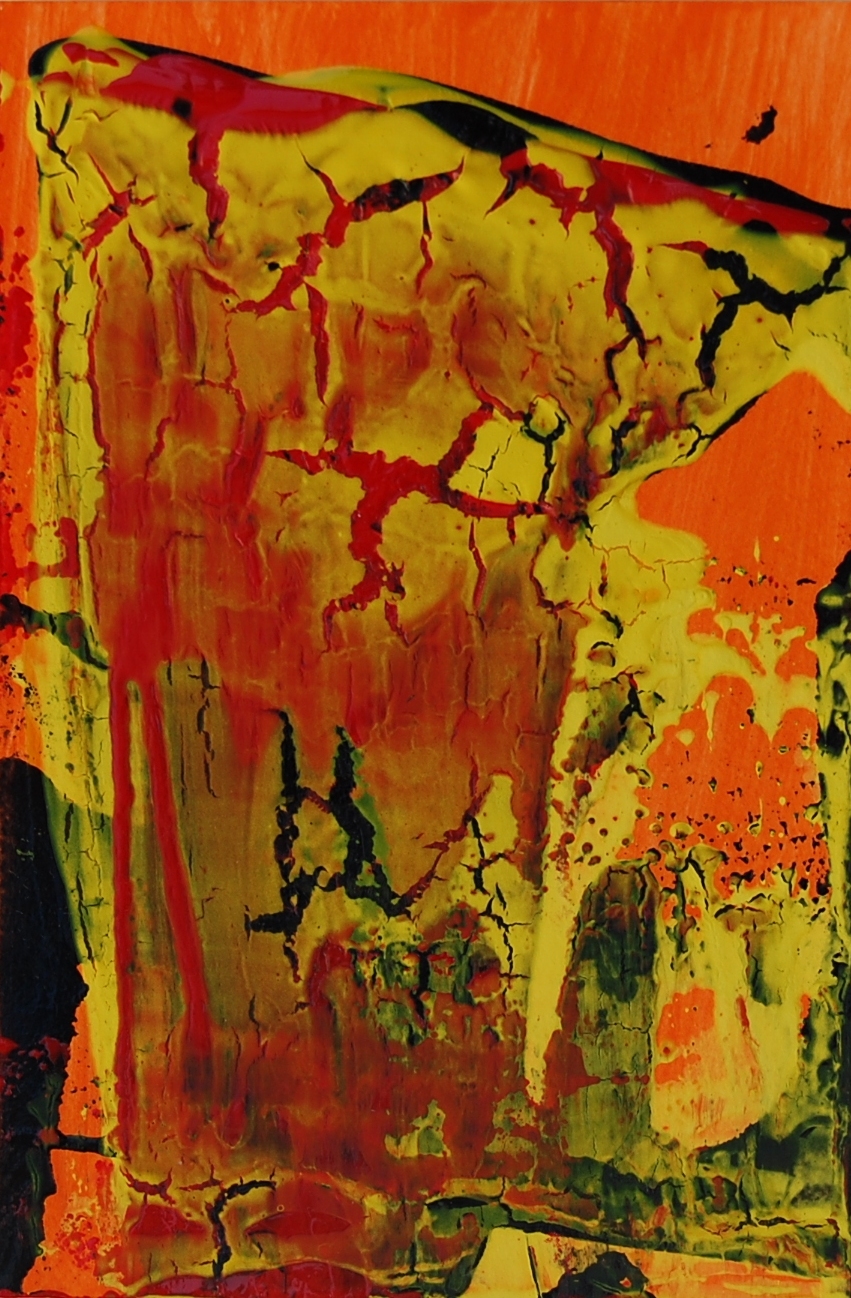This esoteric and abstract painting is a complex collage of colors and patterns, predominantly featuring fiery hues. The piece is visually dominated by rich shades of orange and red, with occasional mustard yellow, green, and black accents adding depth and contrast. The colors exude a sense of violence and intensity, reminiscent of a hellish landscape or a volcanic scene. The painting is textured and cracked, with myriad lines and shapes extending both horizontally and vertically, creating an intricate tapestry that defies easy interpretation. Reminiscent of an ornate Japanese robe in its pattern, the image lacks any discernible figures, text, or specific imagery. Instead, it invokes the viewer's imagination, with possible formations resembling faces or abstract shapes emerging amidst the chaotic yet beautifully orchestrated layers of color and texture.